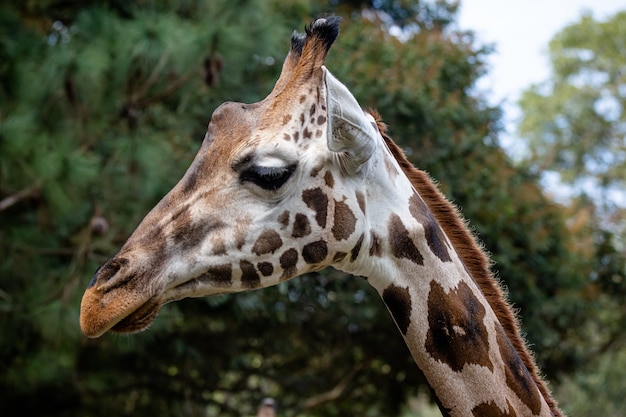The image is a high-quality, vibrant, close-up photograph of a giraffe captured in a horizontal rectangle frame. It shows only the head and part of the neck of the giraffe, which is mainly white with distinctive brown spots and patches. The giraffe is facing towards the left, showcasing its long, triangular-shaped snout with the top lip overlapping the bottom lip and nostrils positioned at the top. Its large, dark eye, accentuated by black markings, stands out, mirroring the black tips of the two small, horn-like protrusions on the top of its head. The ears are almost level with the eye and lighter in color. Additional details include distinctive eyelashes and a slightly wrinkled neck adorned with brown fur running down the mane. The background, while blurred to emphasize the giraffe, reveals a sunny day with a light grayish-blue sky and diverse green trees, providing a natural and serene backdrop.